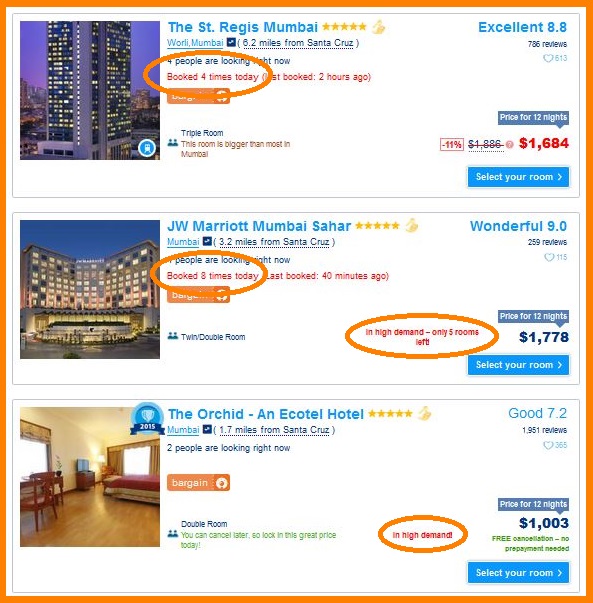This image is a screenshot from an online travel booking website, potentially Expedia, TripAdvisor, or Booking.com. The screenshot features three hotel listings, each with a descriptive layout. Here is a detailed breakdown of each listing:

1. **The St. Regis Mumbai**:
   - **Font and Outline**: The name is displayed in blue font on a white background, with the entire listing outlined in an orange square.
   - **Rating**: It has a rating of 8.8, labeled "Excellent" in blue font, and is adorned with five gold stars.
   - **Photo**: The accompanying image is a night view of the high-rise hotel's exterior, showcasing illuminated windows with a purple-hued sky and some cityscape in the background.
   - **Booking Status**: The phrase "Booked 4 times today" is noted in red font, surrounded by an orange oval shape.

2. **JW Marriott Mumbai Sahar**:
   - **Font and Outline**: Similar to the first listing, the name "JW Marriott Mumbai Sahar" appears in blue font.
   - **Rating**: This hotel is rated 9.0, labeled "Wonderful" in blue, and also features five gold stars.
   - **Photo**: The image presents the exterior of the building, which is slightly shorter and shows a frontal night view.
   - **Booking Status**: It indicates "Booked 8 times today" in red, encircled by an orange oval shape. Additionally, there's a note in orange highlighting, "In high demand, only five rooms left."

3. **The Orchid An Ecotel Hotel**:
   - **Font and Outline**: The hotel name appears with the same blue font.
   - **Rating**: Rated 7.2 as "Good" in blue, with five gold stars.
   - **Photo**: This image features an interior view showing a cozy corner of a room with hardwood floors, beige walls, and furniture in reddish-brown hardwood. There is also a hint of a bed with a maroon bedspread.

The collective design and notation choices, like the orange outlines and ovals, emphasize booking urgency and popularity of these hotels.